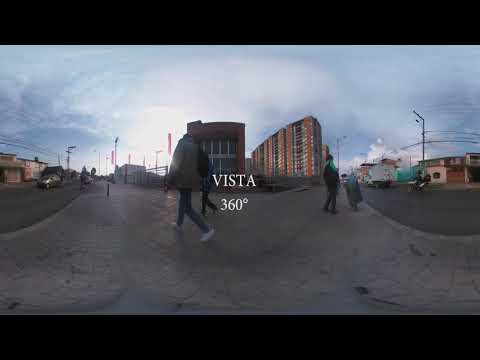In this slightly blurry outdoor image taken from a distance, the focus is on a partly cloudy sky with blue and white tones above a setting that appears both industrial and urban. Centered prominently within the image, there is white text in all capital letters: "VISTA" on the top line and "360 degrees" below it. The scene features two central reddish-brownstone buildings, approximately 10-15 stories high, and additional low-rise structures visible on either side. These buildings flaunt windows with balconies, set against the backdrop of the cloudy sky.

Pedestrians are walking along a light-colored, paved road that splits in the middle, giving depth to the scene. Notable among them is a person donning white sneakers and another with a jacket featuring some green. Scattered throughout the scene are various vehicles, including parked vans, and street lamps, contributing to the bustling urban atmosphere.

The setting also includes power lines and security cameras, indicating a well-monitored area. Although the image's lack of clarity makes it difficult to discern minute details, the overall composition captures a vibrant yet serene urban landscape on a partly sunny day.